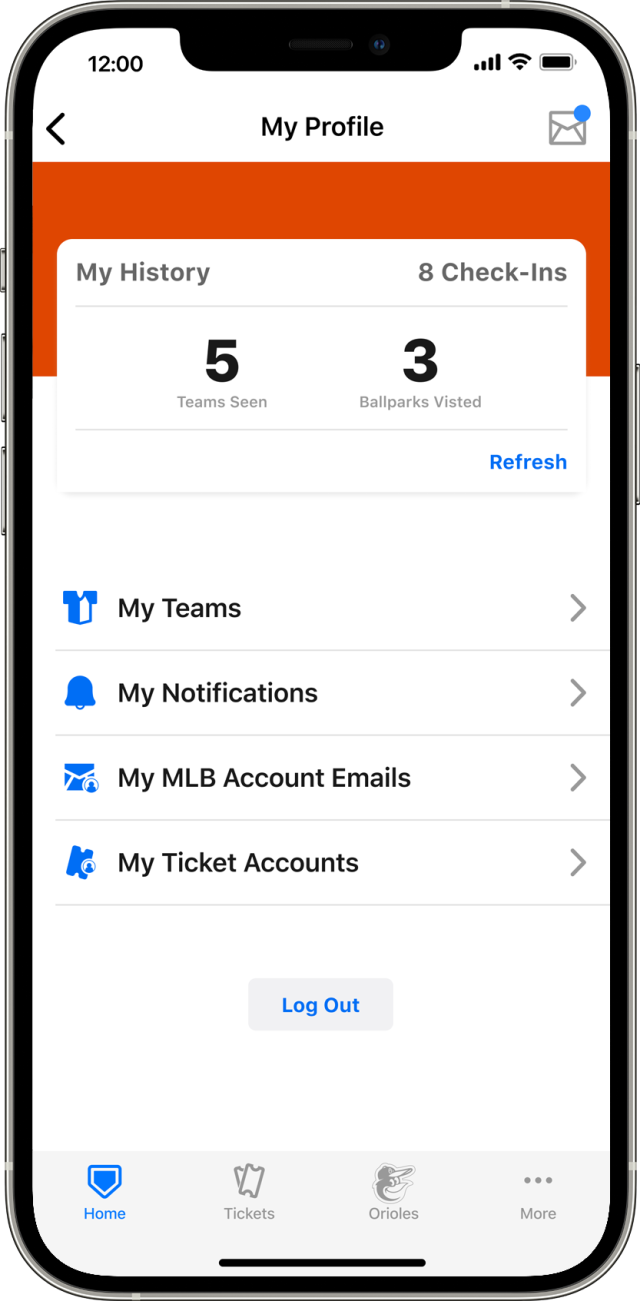In this detailed image, we see an iPhone displaying a specific app interface, likely related to Major League Baseball (MLB) due to the contents and layout. The interface is predominantly white with blue and gray icons, and features a simplistic design.

At the top of the screen, the status bar shows it is currently 12 o'clock, with icons indicating a strong Wi-Fi connection, full signal strength for wireless data, and a fully charged battery. 

The primary section of the screen starts with the title “My Profile” at the top, with a back button to the left and a mail icon to the right marked with a blue dot, suggesting unread messages. Below this, several sections are outlined: 

- **My History**: Reporting 8 check-ins, sightings of 5 teams, and visits to 3 ballparks. A red banner highlights this section.
- **My Teams**
- **My Notifications**
- **My MLB Account Emails**
- **My Ticket Accounts**

Each section seemingly functions as a button to access further details.

Toward the bottom of the app, there is a prominent logout button followed by a navigation bar with options such as Home (currently highlighted), Tickets, an Orioles logo button, and a More button for additional options. The overall clean and user-friendly design makes the application easy to navigate.